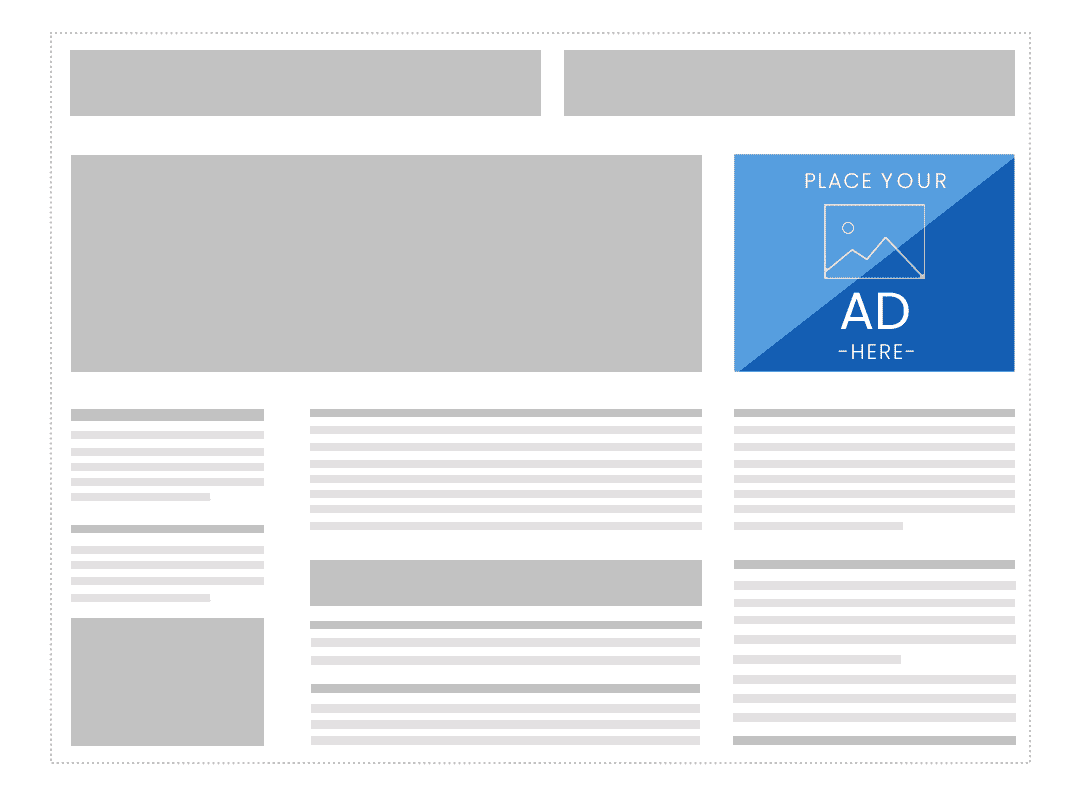A screenshot showcases a structured template for a blog, written document, or website, featuring a predominantly white background with subtle grey accents. At the top, two grey rectangular placeholders sit in a row, followed by a larger, blank rectangular box beneath them. To the right of this larger box, there is a prominent blue square inviting users to "place your ad here." This square is diagonally divided into two shades of blue: light on the top left and darker on the bottom right. Within this blue square is an icon depicting a small mountain with a moon positioned in the top left corner.

Beneath these elements, the template continues with several grey lines arranged horizontally and divided into three columns, likely indicating spaces for text inputs such as paragraphs, blurbs, and write-ups. This layout suggests the template is designed for classified ads or possibly an online newspaper, providing clear guidance on where content can be placed.